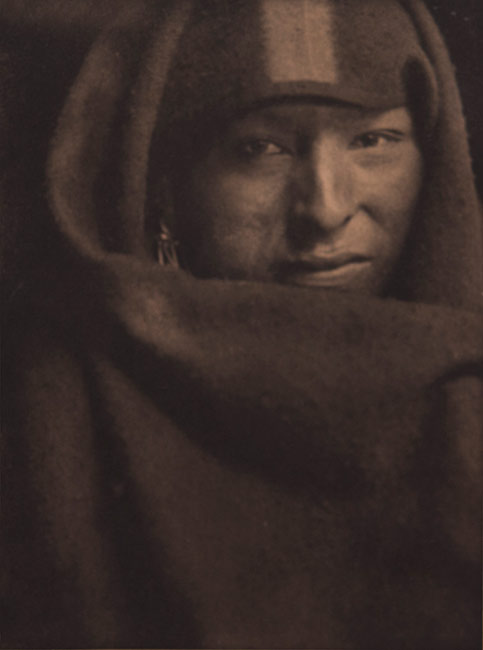The image is a sepia-toned portrait focused predominantly on the face of a person, whose gender is ambiguous, with slightly medium-toned skin. This individual has a very serious, stoic expression with no visible emotions, staring straight ahead with dark brown, almond-shaped eyes. A very dark brown or black fabric is wrapped around their head, covering up to just below the bottom lip and draping over the chest, creating a clean and elegant appearance. Only a portion of the face—from the bottom lip to the eyebrows—is visible, emphasizing the serious demeanor. There is a hint of an earring visible, although the design is not clear. The background is completely black, which further emphasizes the person's intense and focused gaze.